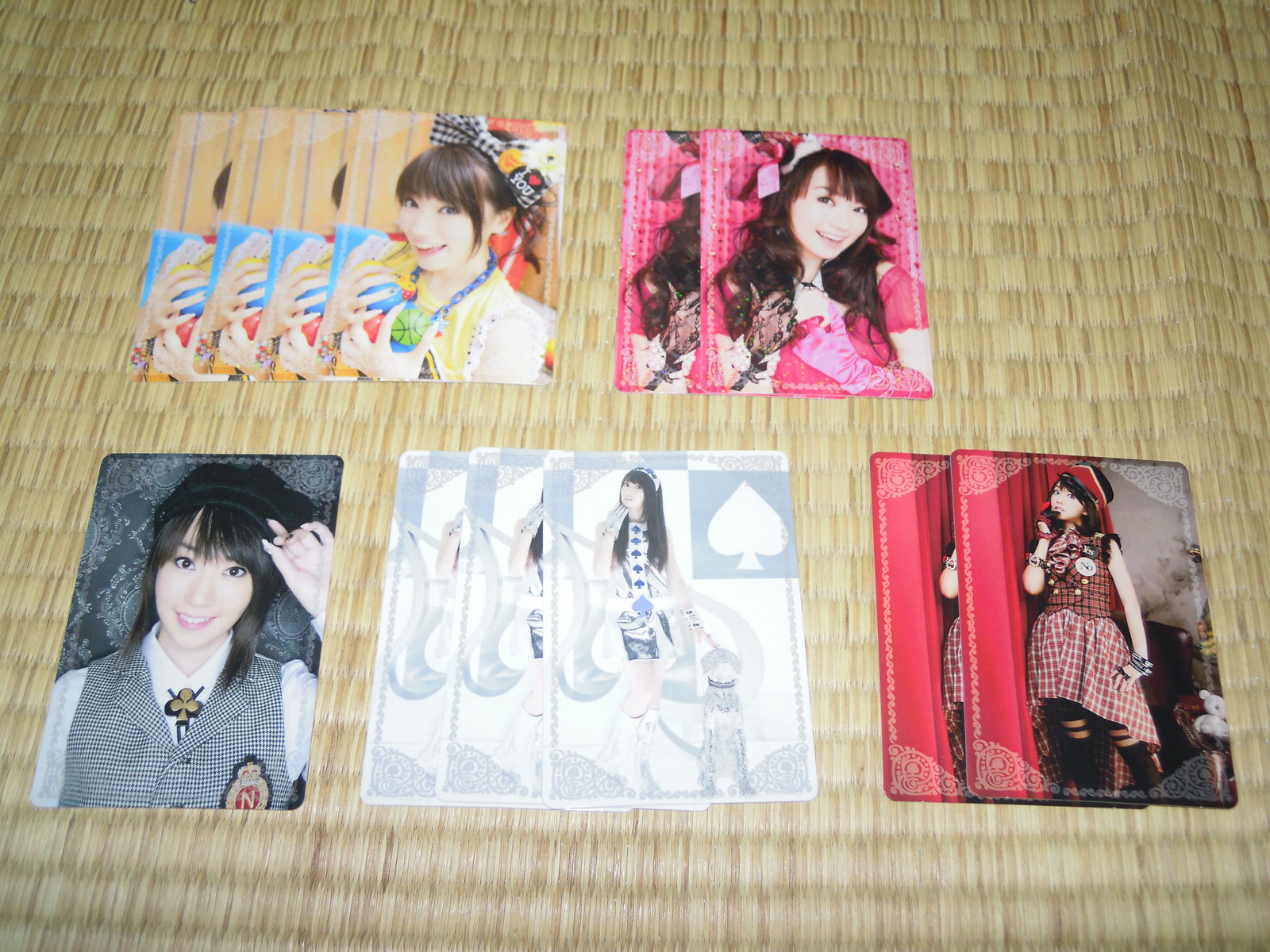This color photograph is taken from an overhead perspective and depicts various piles of fan or celebrity collectible cards scattered on a woven fabric mat, similar to material used in scrolls or window shades, which is brown in color. There are five distinct piles of cards:

1. In the top left, a pile features a girl adorned in ornamental headgear and a decorative necklace, suggesting she is of Asian origin.
2. To the right of this pile, a collection of cards showcases a woman standing and directly facing the viewer, possibly a model. These cards have a peach-colored background in the top left corner and are arranged in a fan shape with four cards overlapping.
3. Below this, there are two cards with a pink hue, also arranged in a fan shape.
4. At the bottom left of the image, a single card displays a woman wearing a white shirt and a checkered blazer, with her fingers touching her hat.
5. In the central bottom section of the image, three illustrated cards feature a woman riding an animal, depicted in a detailed and artistic manner.

Additionally, there's a small pile of two cards showcasing a model standing against a red curtain. The photograph is brightly lit, with the center appearing overexposed, adding a washed-out effect that highlights the central elements of the scene.